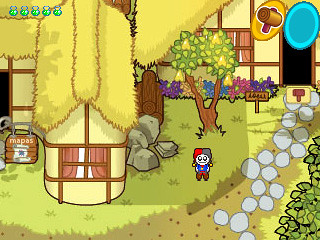Screenshot from the Early to Mid-1990s Video Game: A top-down view captures a character resembling a jester, adorned in red, blue, and grey attire, and displaying a white, smiling face. The scene is set in a village with thatched roofs made of yellow hay, showcasing a distinct European architectural style. Logs are stacked to the side of a hut labeled "mapas" (Spanish for maps). In the background, additional huts line a quaint pathway, completing the immersive look of this nostalgic game environment.